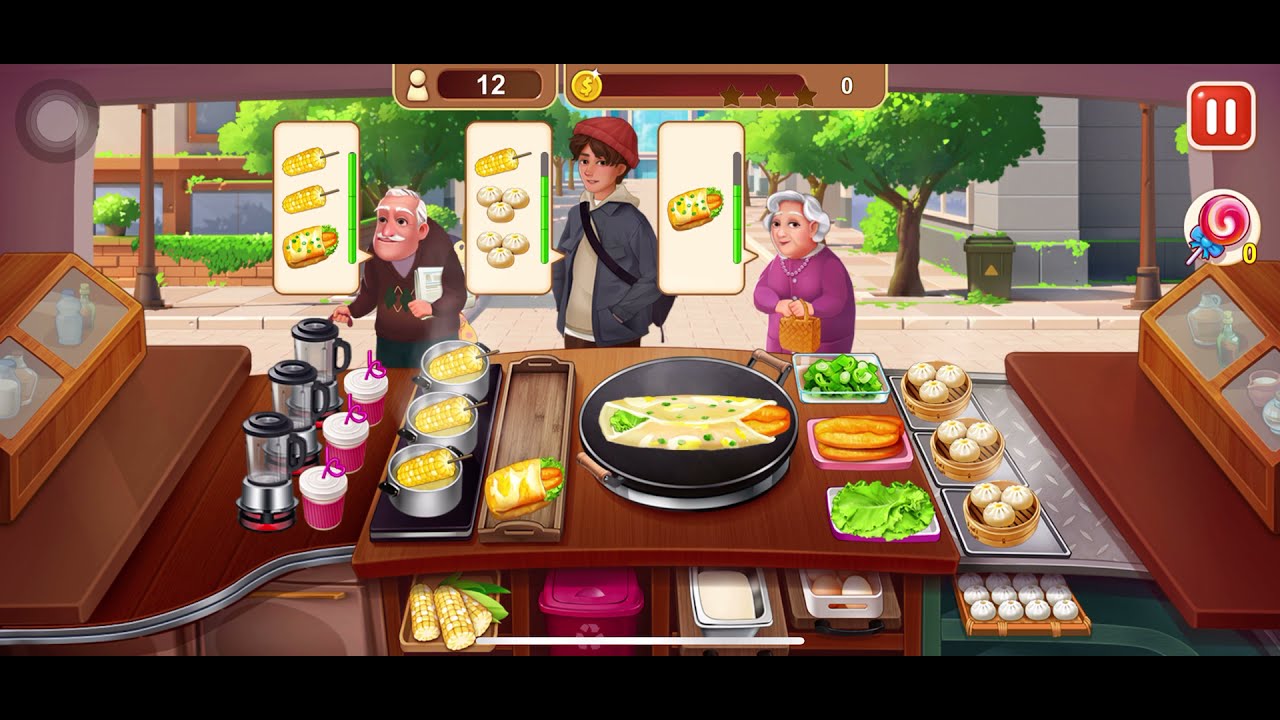This screenshot of a mobile game depicts a bustling restaurant scene with three distinct customers. On the left is an elderly man with white hair and a mustache, dressed in a brown jacket and holding a newspaper under his arm. In the center stands a young boy, sporting a red beanie and a blue overall with a gray shirt underneath, a strap crossing his chest. To the right is an elderly woman, elegantly clad in a purple dress and adorned with a pearl necklace, holding a brown purse.

The scene is set inside a restaurant, viewed from behind the counter. The countertop is laden with various food items and kitchen equipment. Pots filled with corn on the cob, a frying pan with food, and hoagies are prominently displayed. There are also blenders, coffee makers, and containers of green bread, muffins, and tortillas. Ingredients such as onions, lettuce, and other vegetables are organized in compartments. A display case to the right holds additional food items.

Above the characters, a user interface shows a meter with coins and a user icon marked '12'. Adjacent to this, a pause button and a candy cane icon (with the number zero) are visible. Background elements reveal the exterior of the restaurant with a cityscape featuring sidewalks, trees, and buildings glimpsed through the windows.